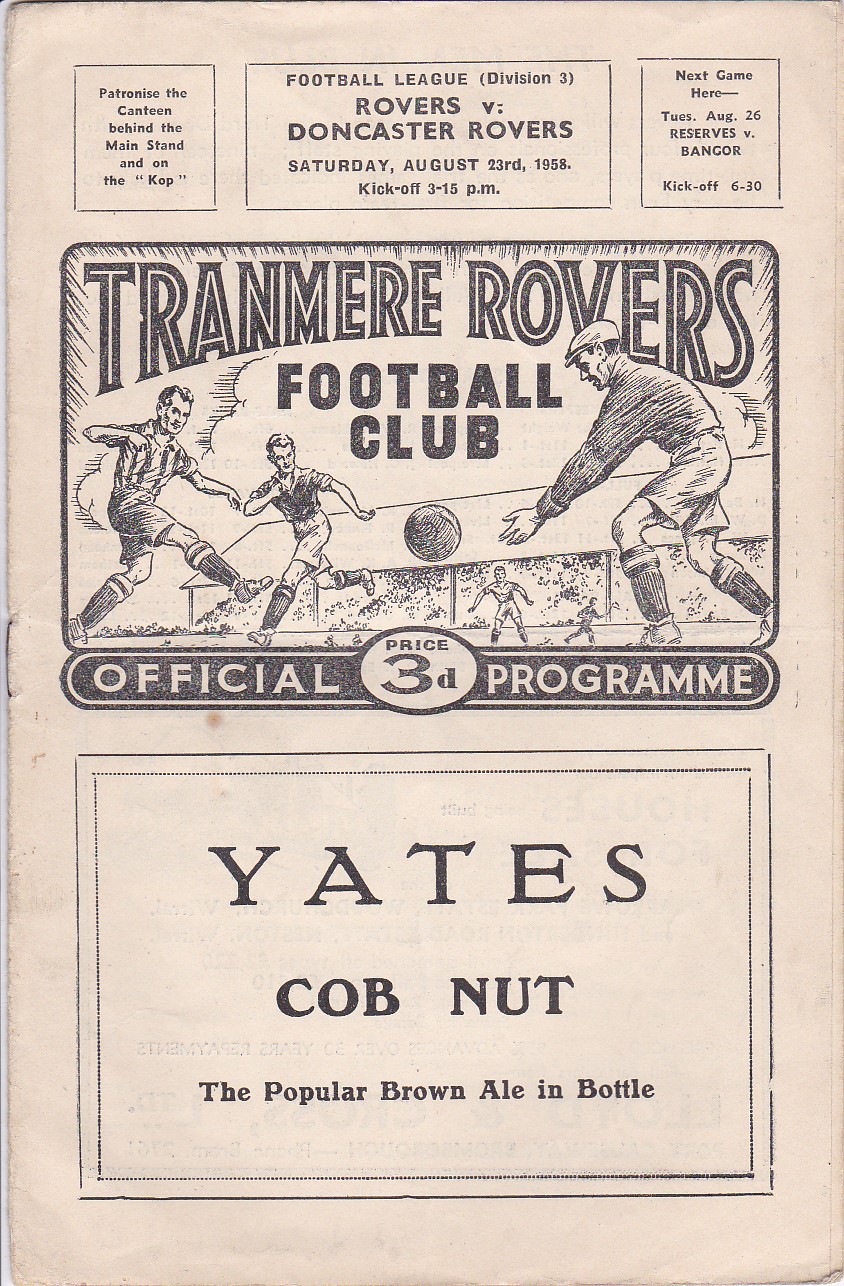The image is a rectangular, vintage football program cover on discolored, aged paper, divided into five outlined sections. On the top, there are three boxes: the first reads "Patronize the canteen behind the main stand and on the KOP." The middle box announces "Football League Division 3, Rovers vs. Doncaster Rovers, Saturday, August 23, 1958, kickoff 3:15 pm." The third box states "Next game here: Tuesday, August 26, Reserves vs. Bangor, kickoff 6:30 pm." Below these, a large rectangle contains a sketch of three men playing soccer with a ball in the middle. Above the sketch, it says "Tranmere Rovers Football Club." Beneath it, the text reads "Official Program" with an inset oval indicating "Price 3D." At the bottom, an advertisement for "Yates Cobb Nut, the popular brown ale in bottle" is displayed.